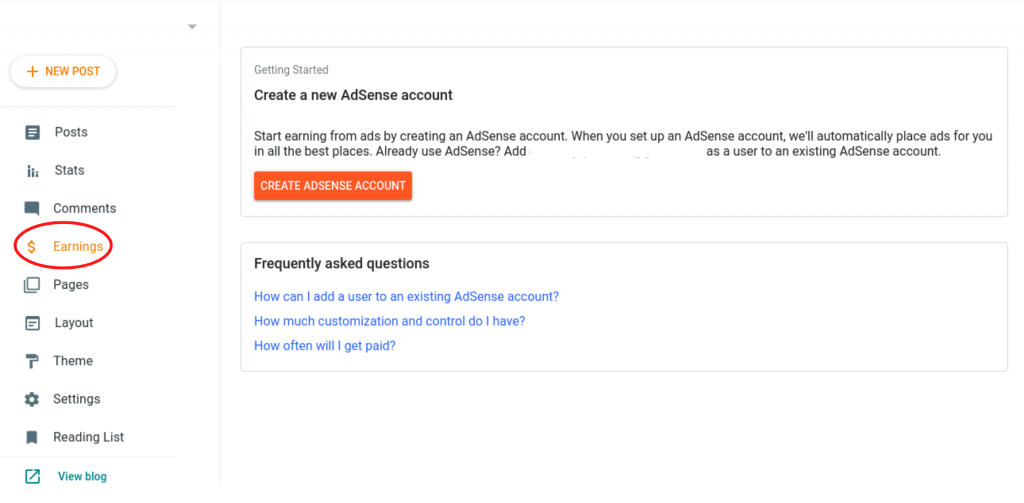The image depicts the back-end interface of a Google AdSense account integrated into a WordPress website. The user interface is predominantly white, providing a clean and simple layout. On the left side of the screen, there is a vertical white sidebar containing 10 menu items: Posts, Stats, Comments, Earnings, Pages, Layout, Theme, Settings, Reading List, and View Blog. Each menu item is paired with an icon to its left and descriptive text to its right.

At the top of the page, there is a prominently displayed, pillow-shaped button in white with orange text that reads "Plus New Post," signaling a quick access point for creating new content. Notably, the "Earnings" menu item in the sidebar is highlighted with a red circle, drawing attention to it. This detail suggests that the user is possibly focused on checking the financial performance or income generated through the Google AdSense platform.